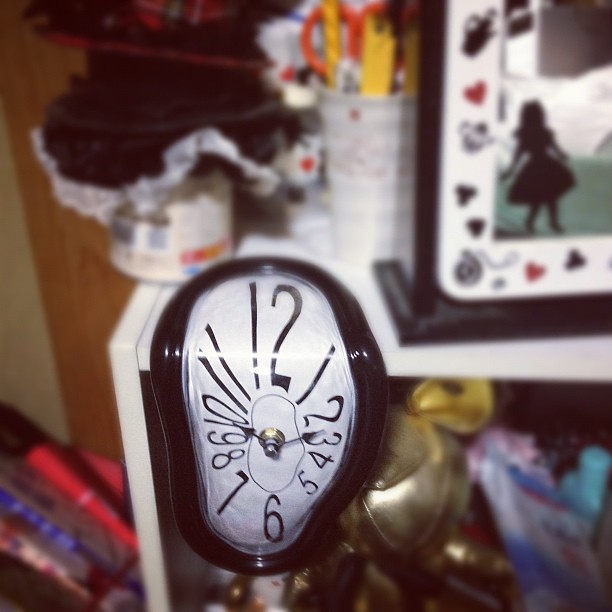This image features a surreal, melting black-framed clock draped over the edge of a white shelf, creating an effect reminiscent of Salvador Dalí's famous works. The clock's distorted face shows the time as 10:12, with creases prominently bending through the numbers 11, 12, and 1. The white shelf, which resembles a cheap bookcase, holds several items, including a brown wooden picture frame with a silhouette resembling an Alice in Wonderland theme, decorated with black and red card suits. Beside it, there’s a cup filled with pencils and a pair of orange-handled scissors. In the background, a cylindrical can topped with a doily and a tan door with dark stains are visible. The chaotic room also includes baseball bats in the corner, and bags of various colors—green, blue, pink, and gold—are scattered on the floor, emphasizing the focus on the melting clock at the center of this eclectic scene.